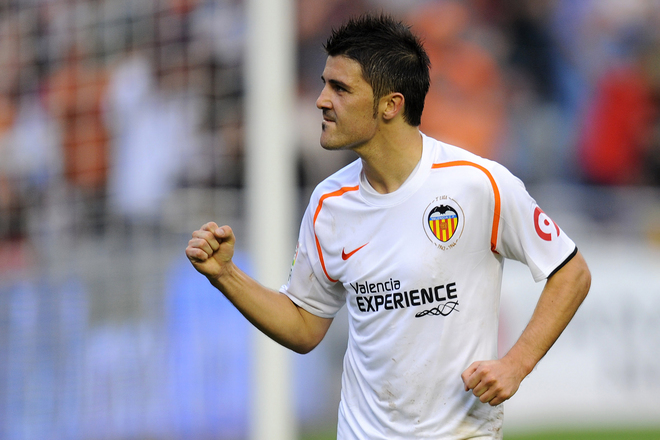The photo captures a moment of triumph for a black-haired soccer player standing by the goal during a game. Dressed in a white team uniform with an orange Nike logo and the words "Valencia Experience" prominently displayed in black text, he exudes a victorious spirit, evidenced by his raised fist. His shirt also features an IMI logo on the chest. The background is a blur of orange, blue, red, and white, likely the colors of fans in the stands, though their details are indiscernible. The black netting and white pole of the goal frame the scene, adding context to the player's exuberant gesture. He sports a barely noticeable mustache, further adding to his distinctive appearance.